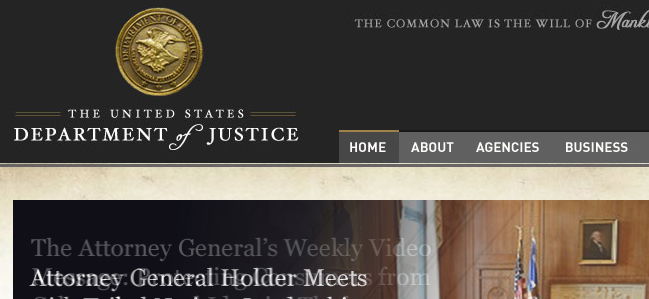The image depicts a dark gray, nearly black background with a gold emblem at the top. This emblem features the Department of Justice insignia, with the text "Department of Justice" written above and below it in white. In the upper right-hand corner of the image, the phrase "The common law is the will of—" is partially visible, followed by what appears to be a cut-off "manK," likely intended to read "mankind."

Beneath the emblem and text, there is a section dominated by four gray tabs. The first tab, highlighted by a brown line, is labeled "HOME" in capital white letters, indicating it is the currently selected tab. The remaining gray tabs, which are not highlighted, read "ABOUT," "AGENCIES," and "BUSINESS."

Below these tabs, the background shifts to a beige color. A prominent rectangle dominates this section, with a gradient that transitions from black to progressively lighter shades. Within this rectangle, two flags are visible, alongside a portrait—perhaps of George Washington or another historical figure.

The text "The Attorney General's Weekly Video" is displayed prominently within this rectangle. Underneath, partially obscured text reads "Attorney General Holder meets..." followed by the visible word "from" and a letter "S," indicating that the full message is cut off by the layout.